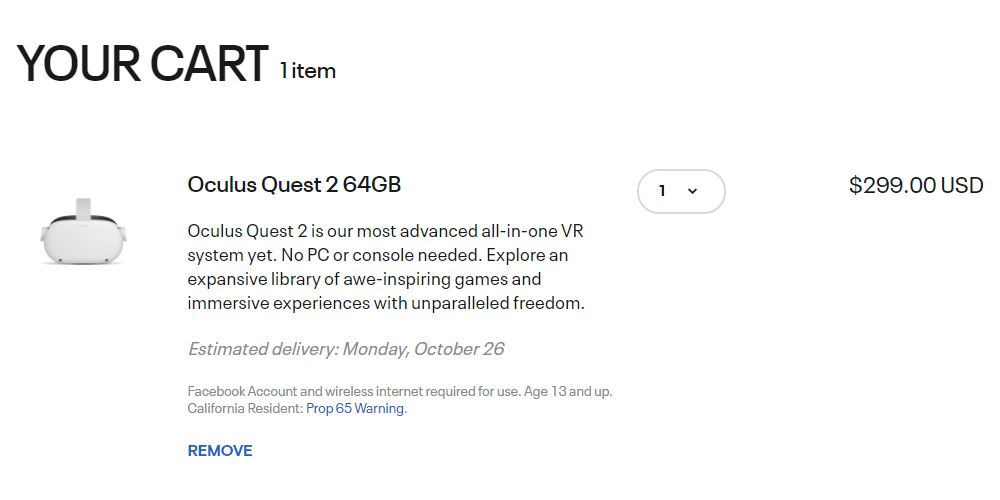**Caption: Oculus Quest 2 Promotional Image**

The image showcases the Oculus Quest 2, prominently displayed as an item for purchase. Below the product, a descriptive tagline reads: "Oculus Quest 2 - Our most advanced all-in-one VR system yet. No PC or console needed." The description emphasizes the extensive library of games and the immersive experiences it offers, highlighting the unparalleled freedom the system provides. It notes the requirements of a Facebook account and wireless internet for use, and specifies the recommended user age as 13 and up, particularly mentioning California residents. The price is clearly marked at $299 USD. A white screen borders the image, offering an option to remove the item from the listing. The product appears to be the only selected item, visually confirmed by a highlighted checkbox or selection mark.